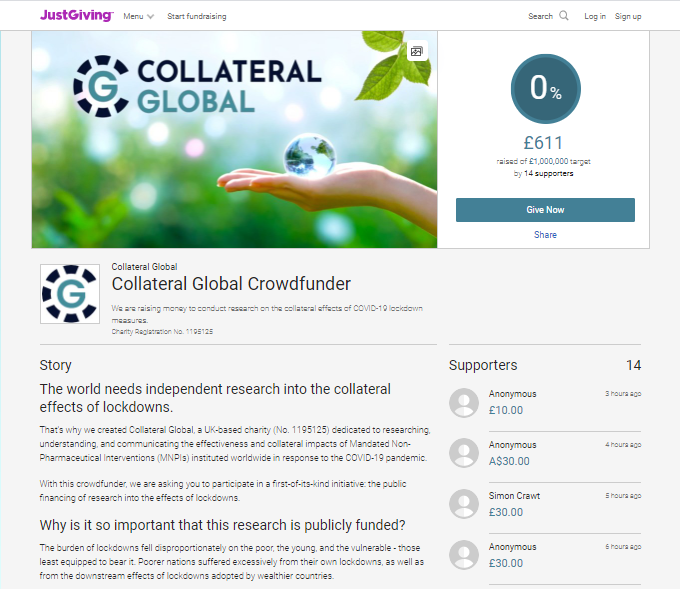The screen capture is from the JustGiving website, featuring a fundraising campaign titled "Start Fundraising." The campaign is led by an organization named Collateral Global, which is appealing for financial support. At the center is an image of a person holding a crystal globe, symbolizing the Earth, in the palm of their hand. 

Collateral Global aims to raise £1,000,000 to conduct independent research into the collateral effects of lockdowns. Thus far, they have raised £611 from 14 donors, which is 0% of their ultimate goal. The campaign highlights the critical need for publicly funded research into these effects, emphasizing the importance of transparency and independence. The details include small text about their story and purpose, along with information about receiving anonymous donations ranging between £10 and £30.